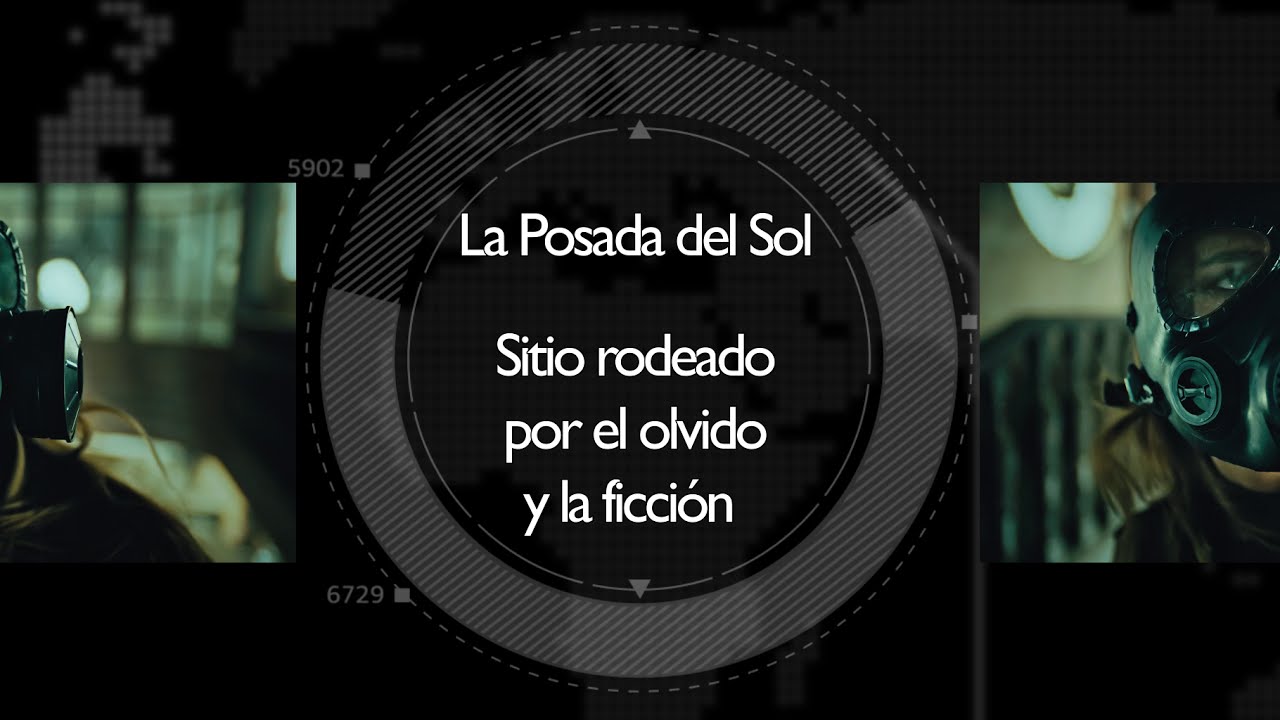The image features a central circular design with a black background and a dotted ring around it, incorporating a striped pattern. The white text within the circle reads, "La Posada del Sol, sitio rodeado por el olvido y la afición." Surrounding the circle, there are numbers positioned in different spots: 5902 is in the top left, and 6729 is in the bottom left. Notably, the right side lacks a number. The image is split, showing a woman’s face divided across the circle. On the right side, the partial image displays the left half of her face, obscured by what appears to be a gas mask or a pilot helmet, with her eye and hair visible. The left side similarly shows the right half of her face, again covered, indicating she is wearing some form of protective gear, possibly related to her occupation.